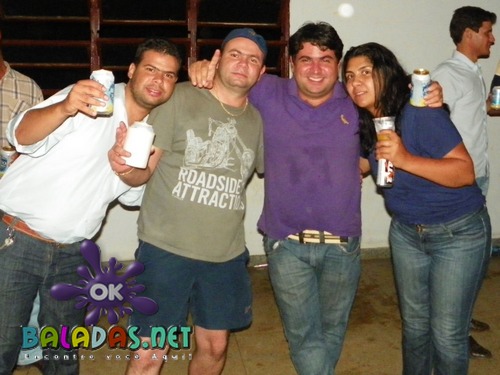In an indoor party setting, four individuals are captured smiling and posing together, holding beer cans. The man on the far left wears a white button-up shirt and blue jeans, leaning towards the group with a cheerful expression. Next to him, a man in a green T-shirt with the print "Roadside Attraction" and blue shorts stands with a beer in his hand, a backward blue baseball cap, and a necklace. His arm is behind the man to his right, who dons a purple polo shirt and blue jeans, appearing slightly sweaty, suggesting it could be warm in the room. This man is placing his arms around both people next to him while raising a finger in the air. The young woman on his right, with long black hair, sports a blue T-shirt and blue jeans, also holding a beer. They all face the camera with smiles, against a backdrop featuring a wooden brown bookshelf and a large window framed with brown, indicating it's nighttime. The room has a cork floor, appearing wet, possibly from spilled drinks.